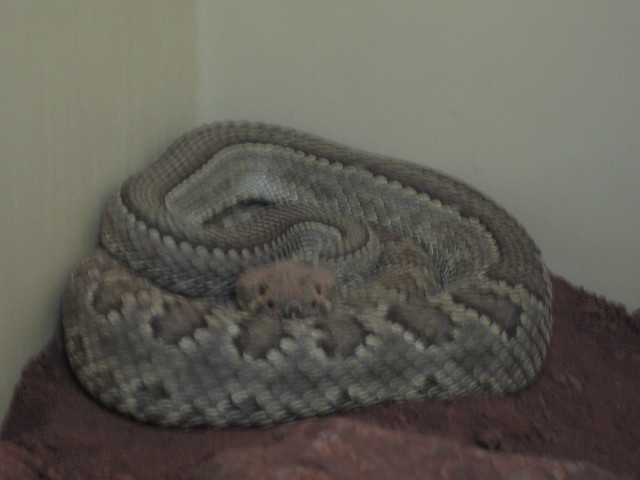The image depicts a coiled-up snake, which appears to be either a rattlesnake or a viper, based on its distinctive diamond-shaped markings and flat, brownish-gray head. The snake is predominantly gray with darker gray, brown, and some off-white earth-toned patterns across its body. It is resting in a tightly coiled position, with its head nestled within the coils, suggesting it could strike at any moment. The snake is set against a reddish clay or dark brown surface beneath it, which resembles a blanket, towel, or possibly dirt. The background consists of off-white walls, giving the impression that the snake is housed in an indoor enclosure, potentially a zoo exhibit or a pet container. The overall setting looks like an angled shot taken from above, highlighting the snake's formidable size and striking markings.